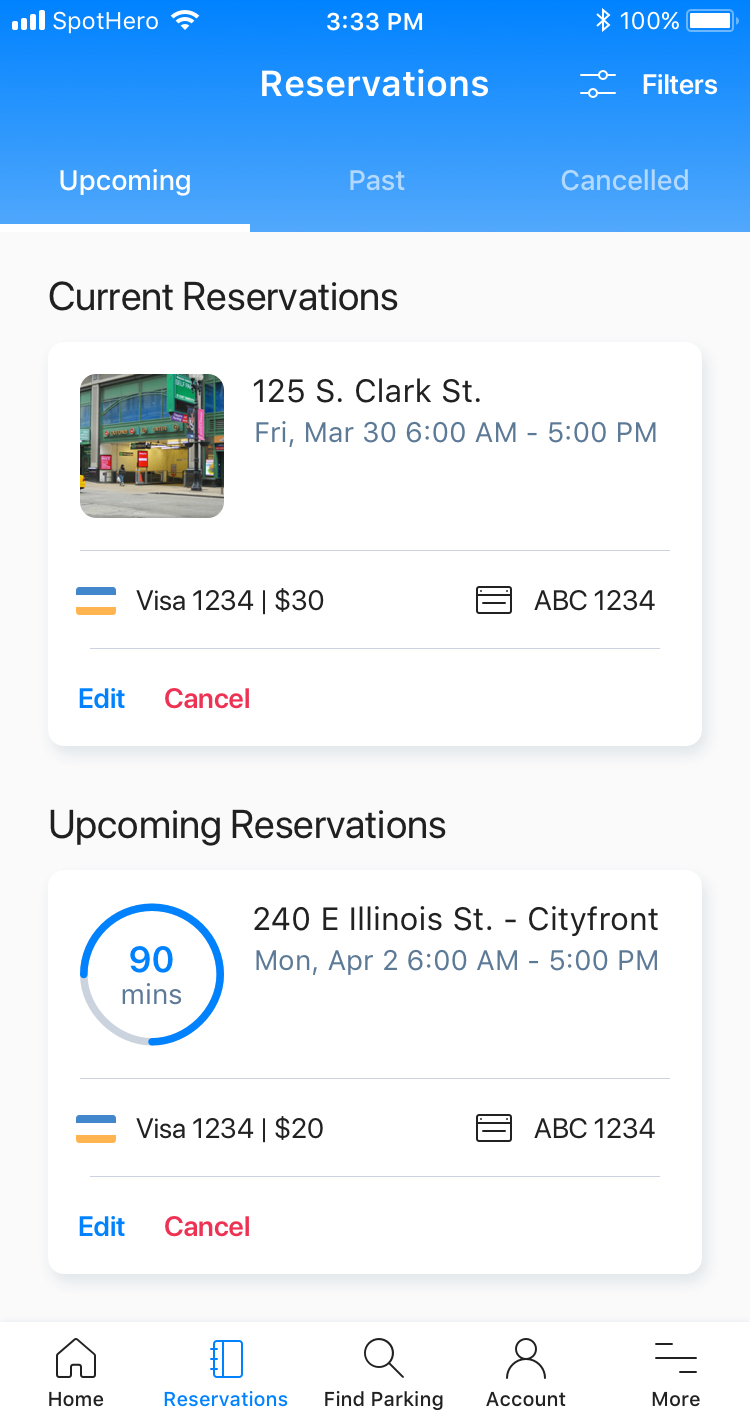The screenshot shows a cell phone display featuring the Spot Hero app interface at 3:33 PM, with full cellular reception, Wi-Fi, Bluetooth, and a 100% battery level. 

At the top center, "Reservations" is prominently displayed, accompanied by a filter icon consisting of two small sliding arrows on the right. Below this, three tabs are visible: "Upcoming" (underlined), "Passed," and "Canceled," set against a gray background with black text indicating navigation options.

Under the "Current Reservations" header on the upper left of a gray background, a white card displays a picture of a building labeled "125 South Clark Street." This card includes a reservation date of "Friday, March 30th, 6:00 PM - 5:00 PM," alongside payment details with a Visa card ending in 123. The amount listed is $30, with options for "Edit" in blue and "Cancel" in black on the right.

Beneath, in the "Upcoming Reservations" section, a blue circle with a gray segment indicating "90 minutes" stands out. It lists a reservation for "240 E Illinois Street, City Front," scheduled for "1:26 PM - 5:00 PM," using the same Visa card ending in 123 for $20. Again, options for "Edit" in blue and "Cancel" in black are available on the right.

Finally, the app's navigation bar at the bottom of the screen includes links to "Home," "Reservations," "Find Parking," "Account," and "More."